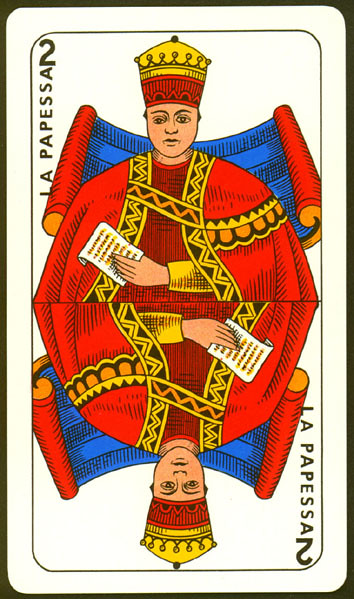The image depicts a tarot card, resembling a traditional playing card but with distinct symbolic details. The card, which is taller than it is wide, is bordered in black. Along the left side of the border, the word "La Papesa" (P-A-P-E-S-S-A) is inscribed, indicating the card's title. The number "2" is positioned above this inscription. 

The card features a mirror-image design with a central figure that appears upright in the top half and inverted in the bottom half. The upper portion showcases a person adorned in a crown and red robes, set against a background of a blue scroll with red edges. The figure's left hand is positioned across their chest, holding a sheet of paper with black writing, which is highlighted in yellow. The visible part of the figure extends from their ribs upward. The lower half of the card perfectly mirrors the top half, presenting the same figure and elements in an upside-down reflection.